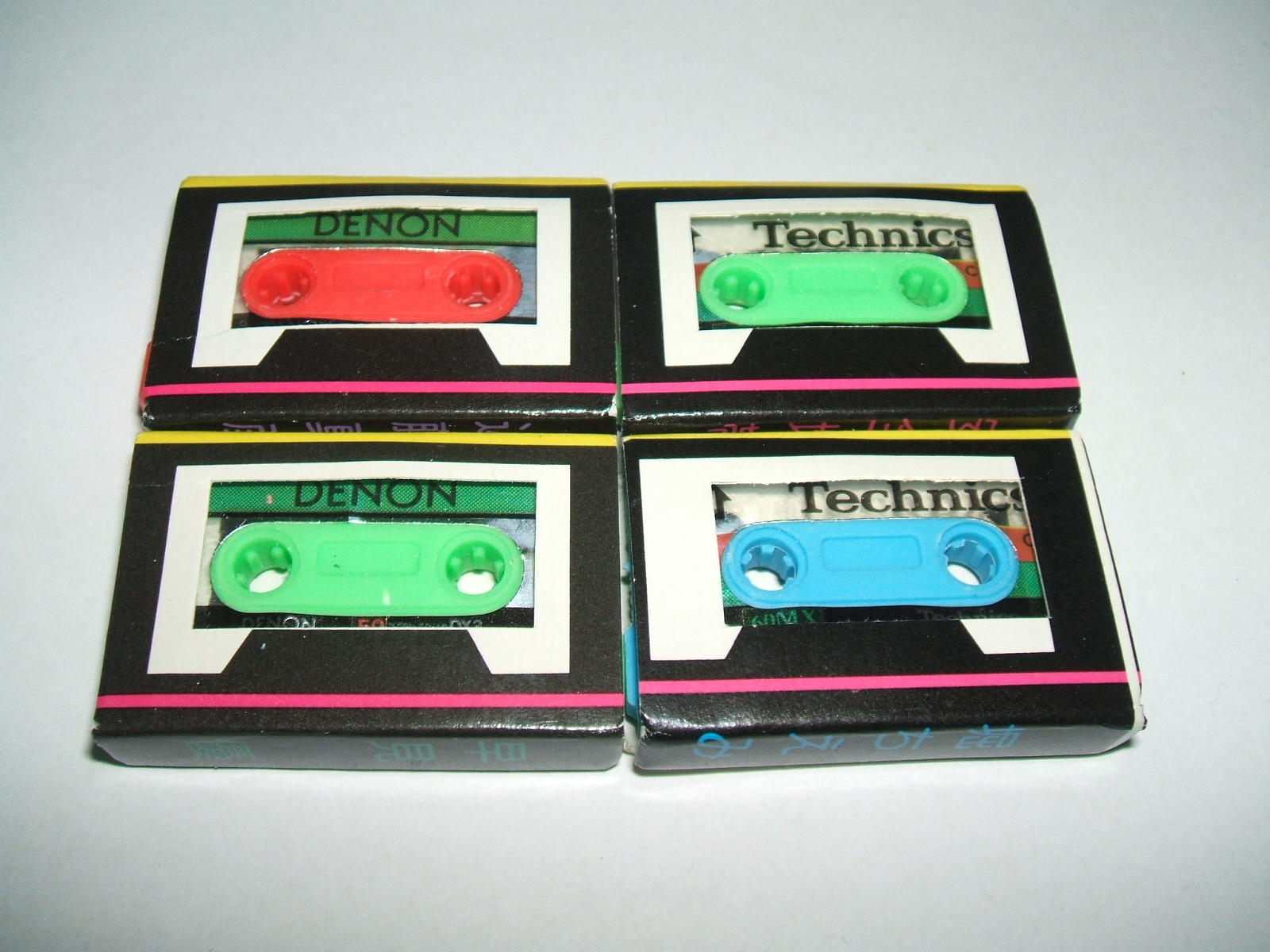This color photo features four vintage-style cassette tapes laid out on a white surface, forming a perfect square. The tapes are arranged in two rows of two: The top left tape has a red take-up reel, the top right has a green take-up reel, the bottom left has a green take-up reel, and the bottom right has a blue take-up reel. Each tape is encased in packaging with a black border, featuring a yellow line across the top and a pink line across the bottom. The tapes on the left are labeled "DENON" with green stripes, and those on the right are labeled "TECHNICS" with white stripes, although parts of the Technics labels are obscured by the plastic gears within the tapes. Additionally, the right-side tapes display faint Chinese characters and the number "200" is visible on the bottom left tape. Despite appearances, these could be novelty items or representations rather than functioning cassette tapes.